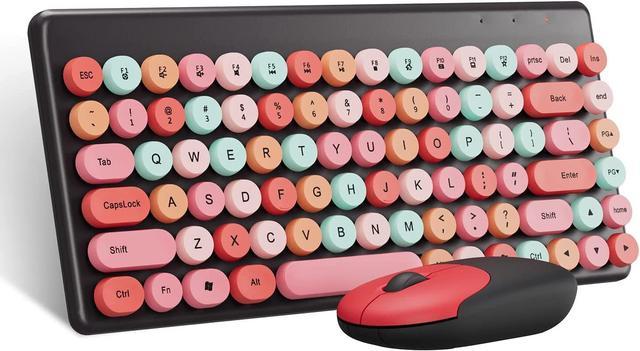The image showcases a unique, colorful wireless keyboard and mouse set. The keyboard features keys in shades of pink, tangerine, and baby blue, set against a dark gray or black base. The keys are all round or have rounded edges, resembling candy buttons or the type of candy found on a candy necklace, giving the keyboard a whimsical, almost cartoon-like appearance. Additionally, the keyboard lacks a number pad and has a Windows key, suggesting it is made for Windows systems. In front of the keyboard sits a matching wireless mouse, designed in black with red accents, maintaining a simple functionality with a right-click, left-click, and scroll wheel. The overall aesthetic is very attractive, unique, and colorful, likely appealing to many people due to its playful design.